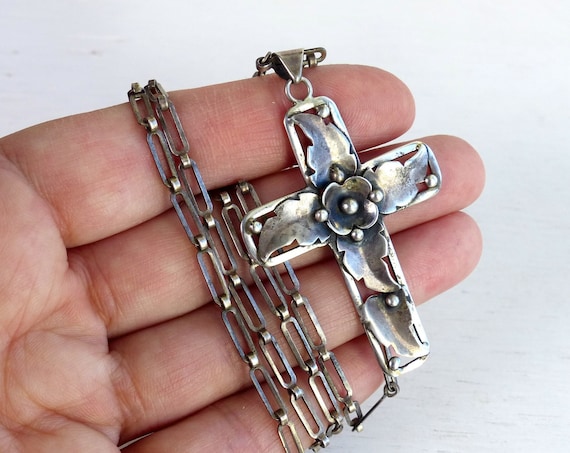This is a close-up photograph of a piece of jewelry, specifically a necklace, centered prominently in a wide vertical rectangular image with a solid light gray background. The necklace features a silver cross pendant adorned with intricate details. The cross is outlined and filled with delicate silver leaves, converging towards the center into a small silver flower, accentuated by tiny silver knobs at the top, bottom, left, right, and the very center. The cross itself measures approximately two inches in length. The silver chain, composed of oblong rectangular links matching the material and color of the cross, is elegantly wrapped around the outstretched fingers of a hand with a light complexion, presenting the palm facing upwards. The chain coils around the four visible fingers, with the cross laid across their tips. The photograph focuses on the hand and the jewelry against the neutral background, highlighting the intricate details and craftsmanship of the silver cross pendant.